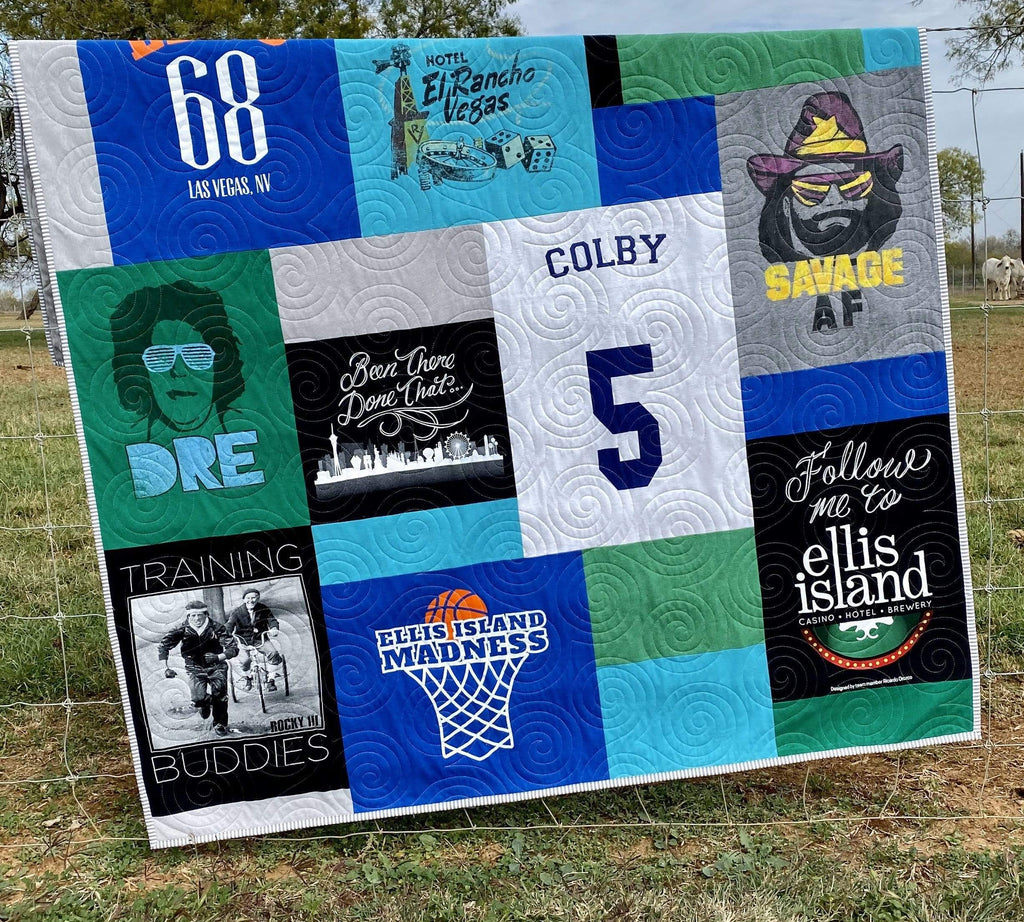The photograph depicts a large, patched quilt draped over a wire fence outdoors. The backdrop features a patchy field of short grass interspersed with patches of dirt, and white farm animals, possibly sheep or goats, are visible in the distance to the right. The quilt itself is an eclectic mix of panels with a variety of themes, primarily focusing on wrestling and sports, but also referencing places and pop culture elements. 

Dominating the quilt is a central white square with "Colby 5" in royal blue text. To its right, there's a depiction of Randy Savage with his iconic cowboy hat and oversized glasses, labeled "Savage AF" in yellow and black. Below this, a black panel reads "Follow Me 2" in cursive, followed by "Ellis Island" in white lettering. Adjacent to this, a blue square showcases "Ellis Island Madness" with a cartoon basketball hoop and ball.

A green panel displays a silhouette of Andre the Giant, marked "Dre" in light blue below his depiction. Above Dre's silhouette, a blue square reads "68 Las Vegas NV" in white, while another square to the left states "Bean There, Done That" in white cursive over a black background with a city silhouette. The topmost light blue square proclaims "Hotel El Rancho Vegas," accompanied by cartoon-style dice and a roulette table.

Additional panels feature "Training Buddies" with a Rocky movie photograph, "Rocky 3," and other phrases like "Casino," "Hotel," and "Brewery." The quilt’s overall color scheme includes dark greens, blues, grays, and blacks, creating a visually rich and detailed tapestry.